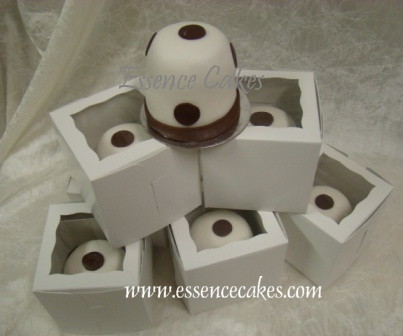This image depicts a stack of intricately decorated miniature cakes. These cakes are nestled in transparent square boxes, which are arranged in a pyramid-like formation on a white tablecloth. The bottom layer consists of three boxed cakes, followed by a layer of two boxed cakes, and topped with an unboxed cake. Each of these delicacies features a white, dome-like form adorned with a chocolate rim at the base and several chocolate candy dots—one on top, and several along the sides. The unboxed cake, resting at the pinnacle, displays the text "Essence Cakes" in faint silver, akin to a watermark. The website "www.essencecakes.com" is prominently written in white text at the bottom of the image, tying the visual details together and revealing that these elegant objects are indeed cakes.